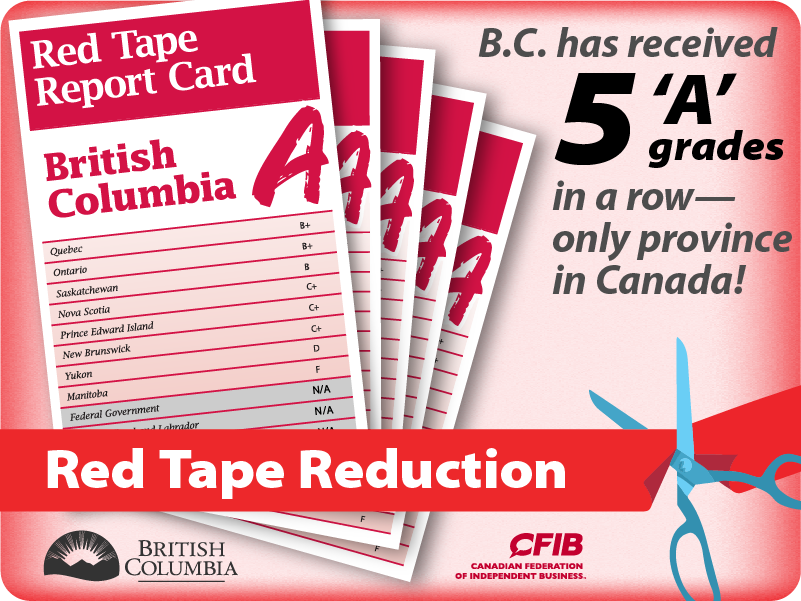This infographic, with a horizontally aligned rectangular shape and curved corners, features a blend of white and red, focusing prominently on British Columbia's exceptional record in reducing bureaucratic red tape. The upper right-hand corner showcases a text highlight that reads, "BC has received 5 A grades in a row - only province in Canada," with '5 A grades' in bold black text for emphasis. The left-hand side displays five vertically stacked report cards with white borders and a red top section inscribed with "Red Tape Report Card." Under each title, there's a white section displaying different Canadian provinces and their corresponding grades: British Columbia proudly holds an 'A', while other regions such as Quebec, Ontario, Saskatchewan, and Nova Scotia have lower grades like B+, B, and C+. Notably, Manitoba has received an 'F'.

Central to the design is a red banner labeled "Red Tape Reduction," appearing to be cut by an illustrated pair of blue scissors, symbolizing bureaucratic cutbacks. The infographic's bottom left corner features the British Columbia logo, while the lower right side includes the "CFIB" logo, indicating the Canadian Federation of Independent Business, the body behind this campaign.

Overall, the detailed illustration and textual elements work together to underscore British Columbia's sustained excellence in reducing bureaucratic red tape, celebrating their unique achievement with a visually engaging and informative presentation.